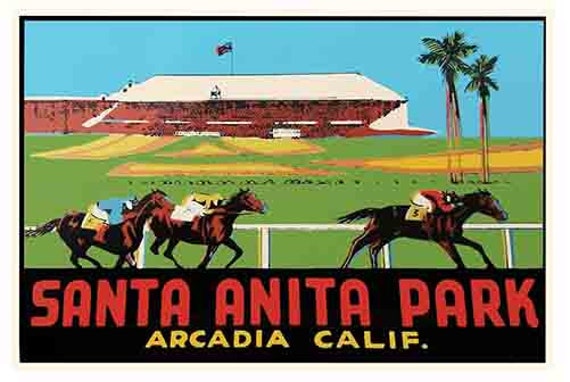The image is a detailed illustration in a nostalgic, old-time postcard style, depicting an exciting horse race with three brown racehorses galloping from left to right along a white-fenced track. The leading horse, marked with the number 3 in yellow, is ridden by a jockey wearing a red top and white trousers. Following closely behind are two other brown horses; one jockey wears a yellow outfit, and the other is dressed in blue. In the background, a lush green field with patches of yellow blossoms spreads out, bordered by two vibrant palm trees on the right. A striking stadium with a sloping white roof and red-painted walls stands majestically, flying a flag atop it. The bright blue sky completes the scene. At the bottom of the illustration, bold red block letters declare "Santa Anita Park," with "Arcadia, Calif." written in smaller, yellow letters underneath.